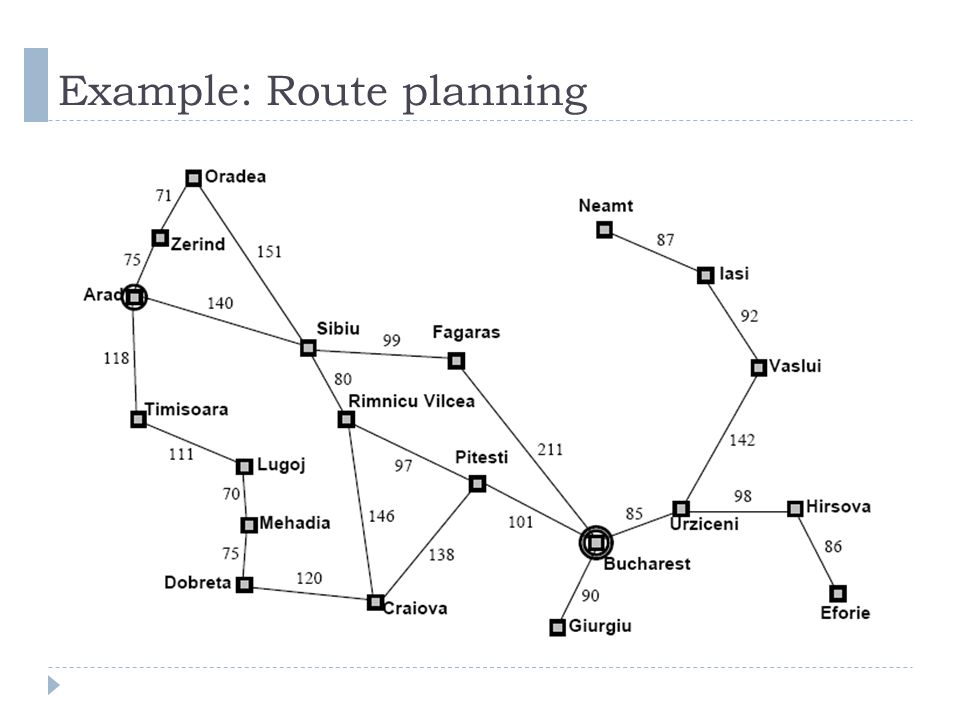The image is a detailed, black-and-white infographic titled "Example Route Planning," displayed on a light blue bar at the top. Below the title, a schematic map in shades of black and gray showcases a network of interconnected locations and distances. Each location is represented by a black square with a gray center, linked by lines that trace possible routes. The locations include Oradea, Zirind, Arad, Timisoara, Lugoj, Mahadia, Dobreta, Craiova, Piatesti, Rimicu, Vilcea, Sibiu, Varagas, Gyorgyu, Bucharest, Erzinceni, Kirosova, Ifori, Vesli, Lassi, and Nemt. The numbered distances between these points range from 21 to 211. Beneath the schematic map is a small light blue dashed line, and a small blue arrow is located in the bottom left corner. The diagram appears to illustrate route planning, potentially indicating distances and connections between different cities or regions.